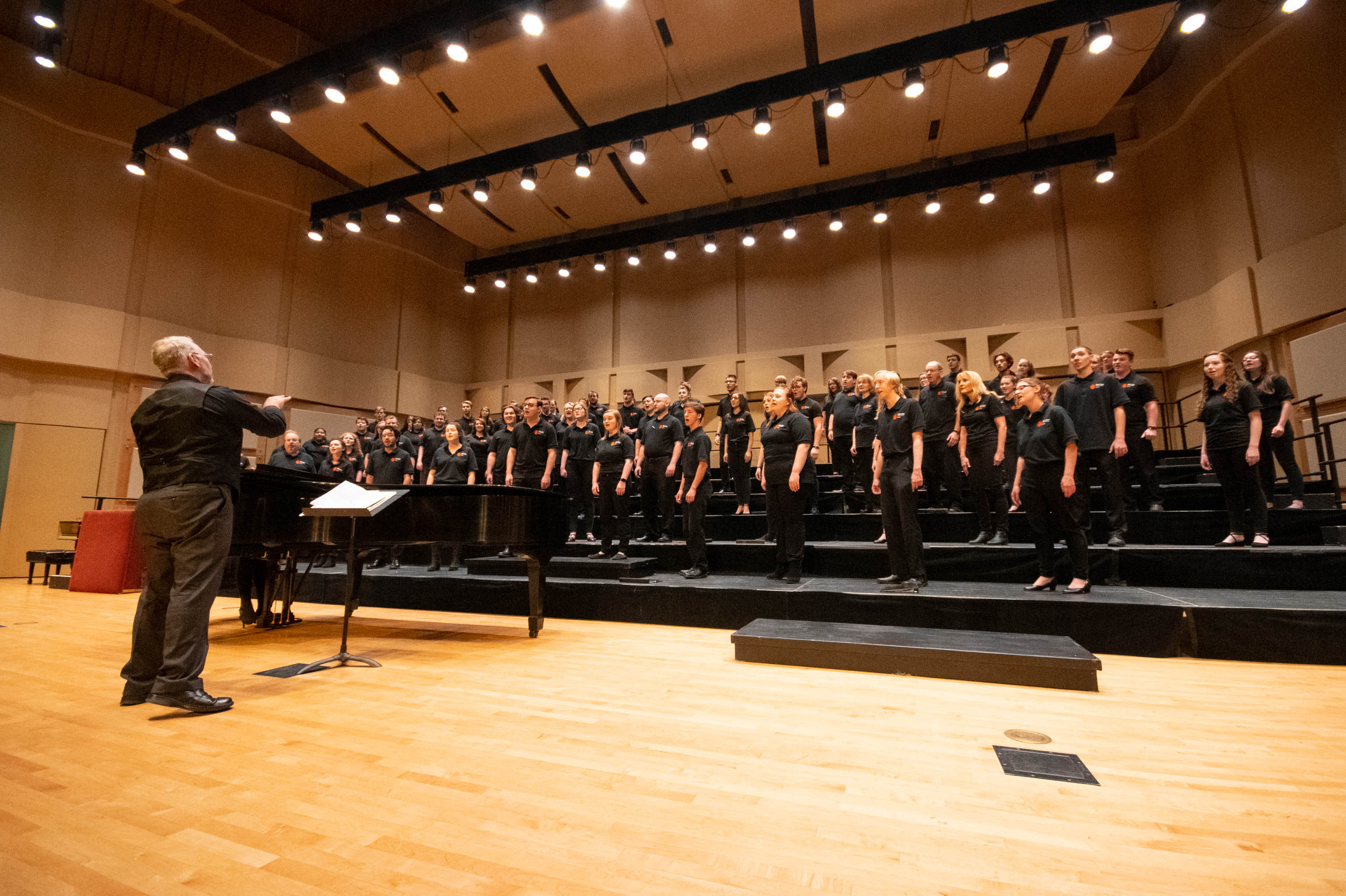The image captures a choir performance in an auditorium-like music room. The choir members, consisting of both young adults and older individuals, are arranged on black, tiered standing platforms that rise gradually, allowing everyone to be visible. All choir members are uniformly dressed in black t-shirts, black pants, and black shoes. Above them, numerous stage lights illuminate the scene. 

Positioned on the wooden stage floor in front of the choir is the conductor, who appears to be an older man with whitish-gray hair and glasses. He is actively conducting with one hand raised, a music stand with open sheet music positioned in front of him. The conductor is attired in a long-sleeved black shirt, dark brown or gray pants, and black shoes. A piano is also visible near him. The overall atmosphere suggests a formal performance that is taking place, although no audience members are visible in the image.